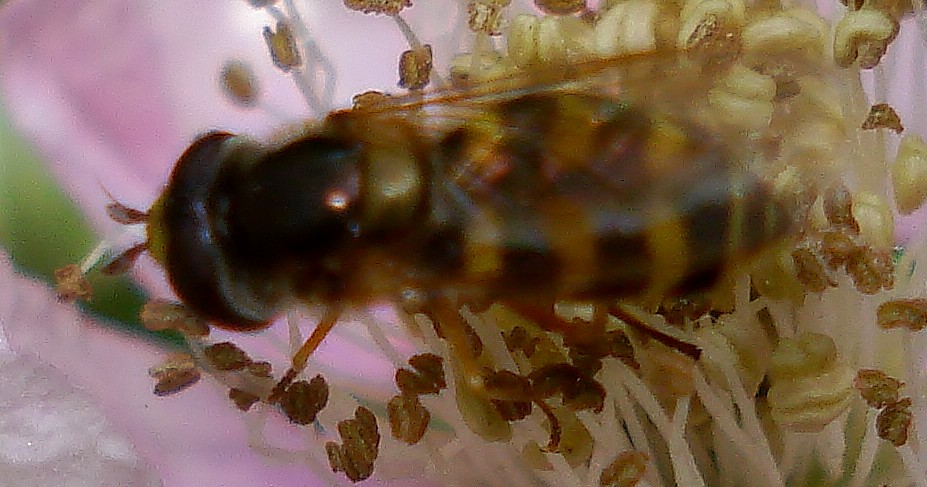The image captures a close-up shot of a bee, taken from above, focusing on its intricate details. The bee, with its black and yellow striped ovalish body, is perched on the interior of a pink and off-white flower. Its body features a shiny, rounded head with yellow at the top and two antennae extending forward. Four thin, yellowish legs are visible, along with its set of transparent, gauzy wings that contribute to the slight blur in the image. The flower's interior is densely packed with small, thin, white filaments tipped with yellow and brown pollen, and stamens are noticeable as well. The background includes a blurred green leaf, enhancing the depth of field in this well-lit photograph.